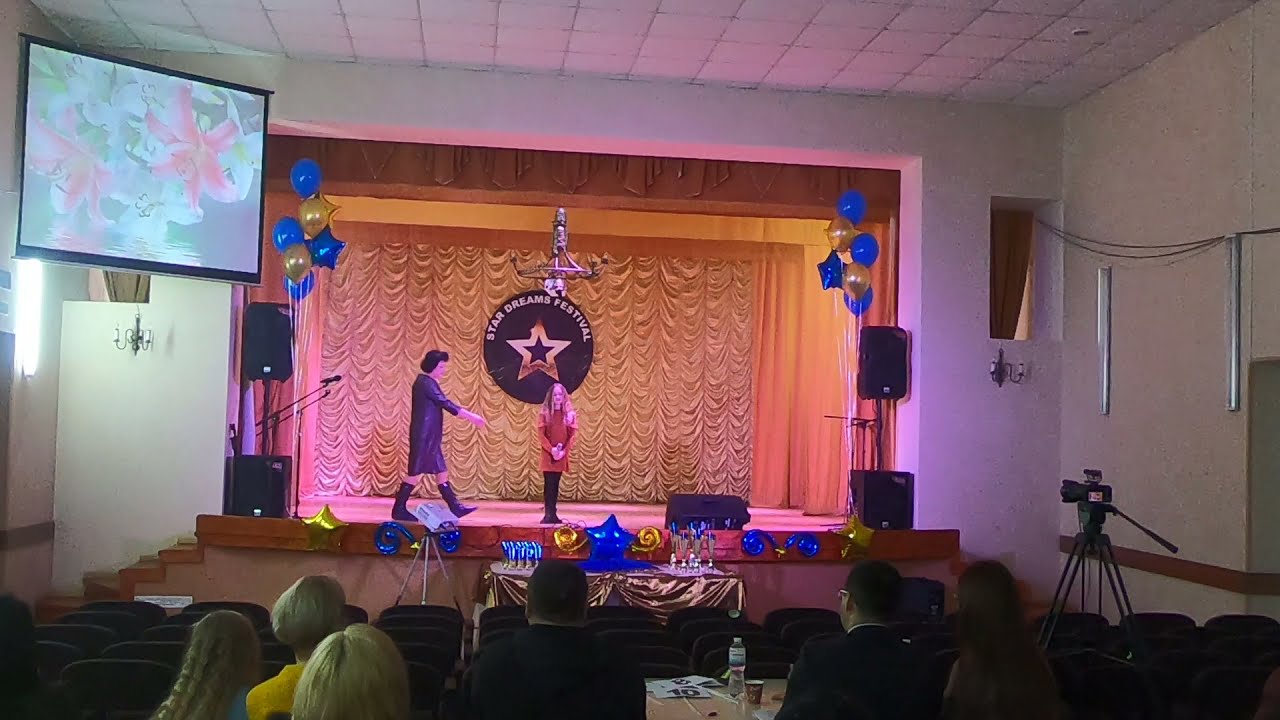The image captures a lively scene at the Star Dreams Festival, taking place on a stage decorated with blue and gold balloons and curtains that frame the backdrop. Centered on the stage, a young girl with long blonde hair stands confidently, dressed in a red long jumper top, black leggings, and boots. To her left, a woman in a black leather dress and matching boots appears to be approaching, contributing to the dynamic atmosphere.

Behind the girl, a large black circle decorates the backdrop, inscribed with "Star Dreams Festival" in white text and featuring a gold star in the center. The stage setup includes speakers and a microphone, indicating preparations for performances. Overhead, a light illuminates the scene while a teleprompter on the left side displays images of pink and white lilies, adding a touch of floral elegance.

In the audience, visible heads suggest a modest gathering, perhaps around six viewers, some of whom seem to be judges. This is inferred from the white signs with black numbers, including an eight and a ten, hinting at an evaluative component to the festival. A video camera in the foreground further enhances the impression that the event is being recorded or broadcast.